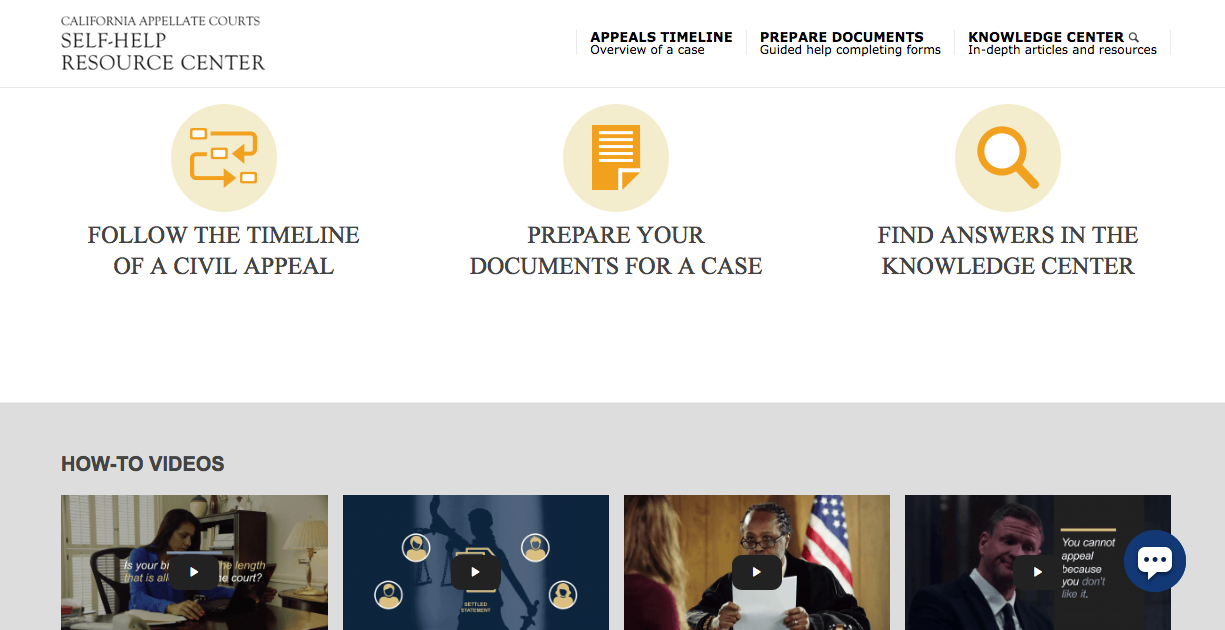This is a cropped screenshot of the California Appellate Courts Self-Help Resource Center webpage. The website features a white background with a minimalistic design and categorizes essential resources into distinct sections. At the bottom, there is a section showcasing four how-to videos; however, their captions are cut off in the image. One video depicts a person at a laptop searching for information, another shows an individual standing before a judge who is reading a document, among other scenes. The website includes various links such as "Follow the Timeline of a Civil Appeal," "Prepare Documents for a Case," and "Find Answers in the Knowledge Center." This resource is specifically tailored for individuals who are navigating the appeals process, providing advanced guidance and necessary information for those who have already undergone initial court proceedings.